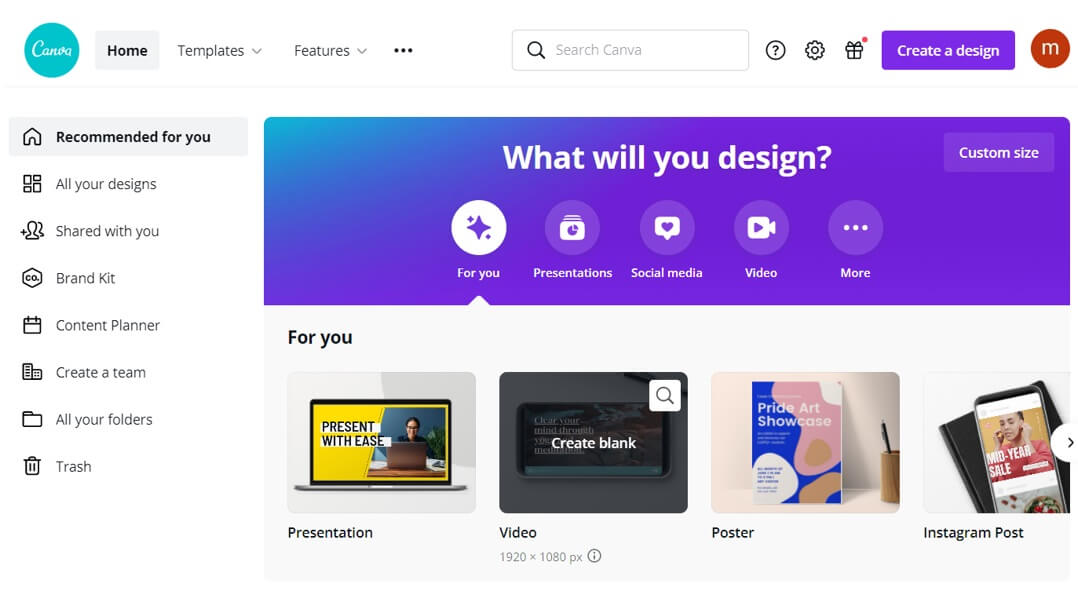The image is a detailed screenshot from the Canva website interface. At the top left corner, there is a small turquoise circle with the word "Canva" in uppercase letters. To its right is a light gray square with the word "Home" printed in black. Adjacent to this are the options "Templates," "Features," each with a downward arrow indicating a dropdown menu, and a set of three horizontal dots symbolizing more options. Also visible is a search bar labeled "Search Canva," alongside icons including a question mark in a circle, a gift box, and a purple banner reading "Create a design."

On the right side, there is a small burnt orange circle with an “M” inside, denoting a personal or profile icon. Below this header section, a vertical sidebar lists various options: "Recommended for you," "All your designs," "Shared with you," "Brand kit," "Content planner," "Create a team," "All your folders," and "Trash."

Dominating the main section of the screen, there's a large purple gradient banner that fades from blue to a darker purple, which prominently features the text, "What will you design?" Below this banner are several circular icons featuring different categories, such as "For you," "Presentations," "Social Media," "Video," and "More." Attached to the purple banner is an additional smaller banner offering a "Custom size" option.

Under these icons, within the "For you" category, options like "Presentation," "Video," "Poster," and "Instagram posts" are presented, presumably suggesting templates or design projects frequently used or recommended based on user activity.